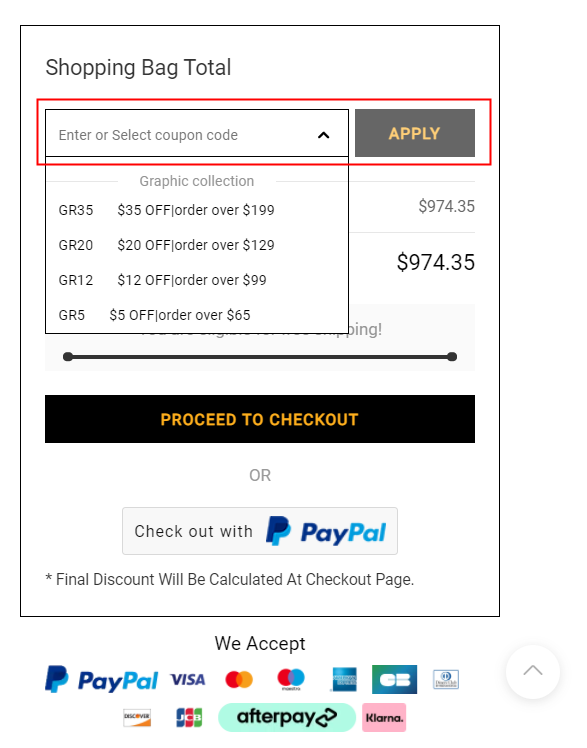A vertically oriented rectangle with a black border displays various informational elements related to a shopping cart and discount coupons. At the top left corner, the text "Shopping Bag" is prominently displayed. Directly below this text is a dropdown menu labeled "Enter or select coupon code," accompanied by an "Apply" button featuring yellow text on a slate gray background. This section is highlighted by a red rectangle, presumably added via a photo editing tool.

Beneath the coupon section, a list of discount codes and their conditions is presented:
- GR35: $35 off orders over $199
- GR20: $20 off orders over $129
- GR12: $12 off orders over $99
- GR5: $5 off orders over $65

A black line with dots on either end demarcates the end of the discount section, aligning with the dropdown menu at the top. Within the same black rectangle, the total amount of $974.35 is displayed twice in succession.

Further down, a large button labeled "Proceed to Checkout" stands out with yellow text on a presumably black background. Adjacent to it is another button, "Checkout with PayPal," which is rendered in two shades of blue and includes the iconic PayPal logo featuring the interlocking "P" design.